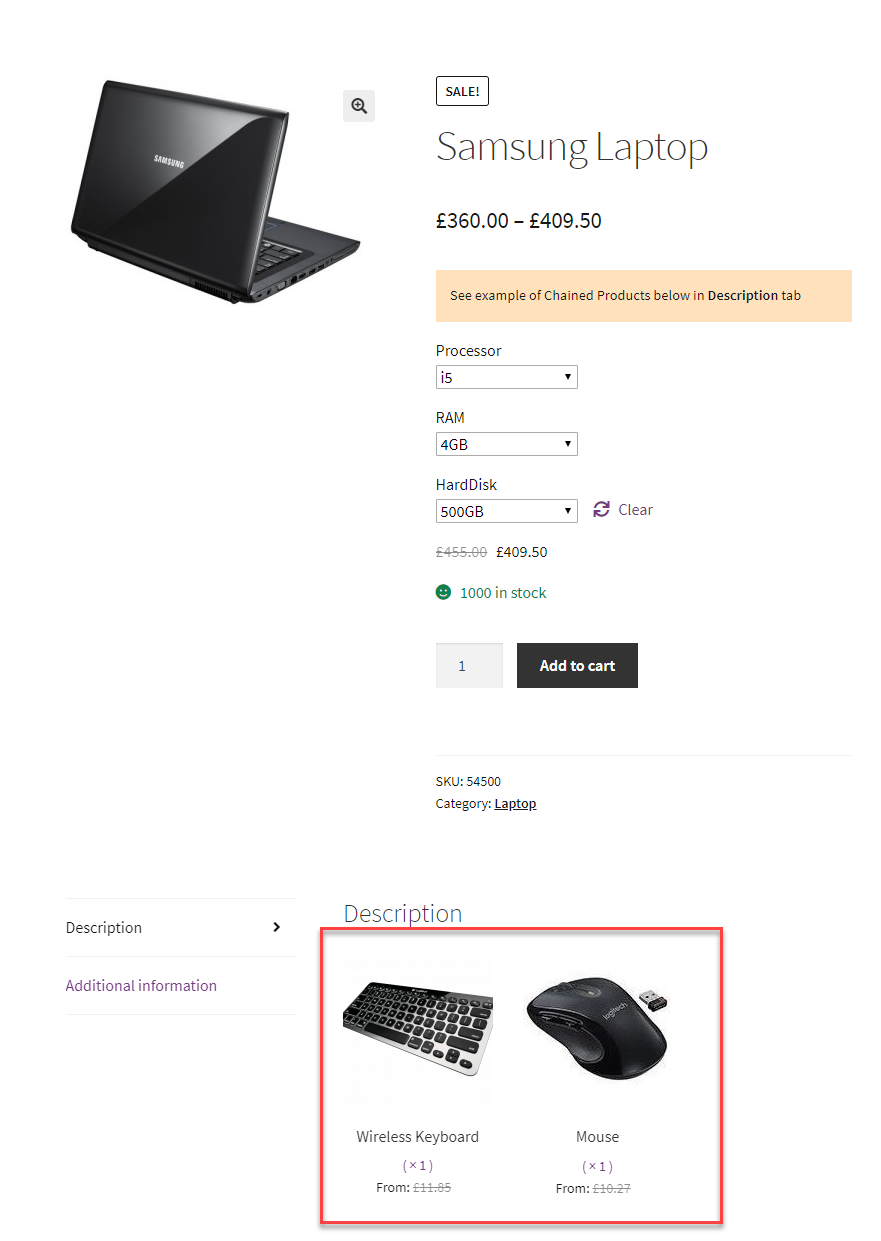A detailed and cleaned-up caption for the image could be:

"The image is a screenshot featuring a black Samsung laptop available for sale. On the left side of the screen, the laptop is positioned with its back facing the viewer, prominently displaying the Samsung logo. Only a small portion of the keyboard is visible. To the right, a black box with the word 'Sale!' in white text draws attention. Below that, the listing reads 'Samsung Laptop' with a price range of £360 to £490.50. The exact currency symbol is not immediately recognizable. The description advises viewers to 'see examples of changed products below the description tab.' The processor type listed is IS, with a dropdown menu for alternative processor options. The laptop comes with 4GB of RAM, which is also configurable via a dropdown menu, and a 500GB hard disk, again with adjustable options. The laptop’s fixed price is stated as £409.50, and there are 1,000 units available in stock."